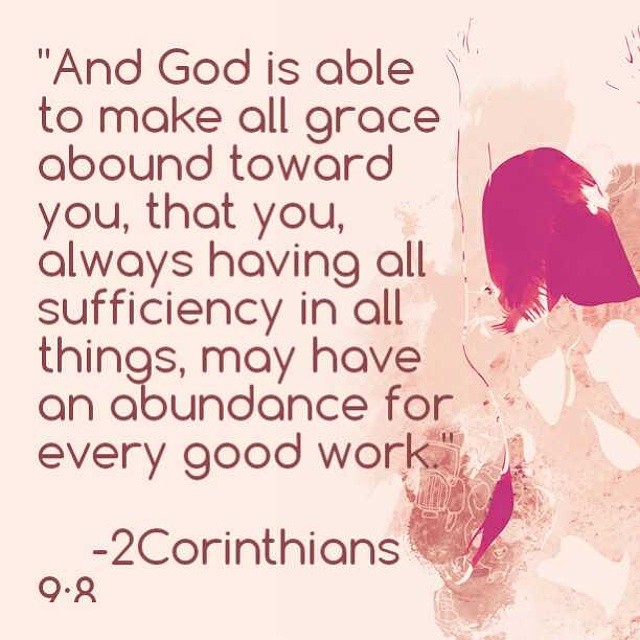The image depicts a poster with an inspirational Christian theme, featuring a quote from 2 Corinthians 9:8. The background of the poster is a blend of light pink hues, whereas the text itself is inscribed in a brownish-red font. The Bible verse prominently displayed reads, "And God is able to make all grace abound toward you, that you, always having all sufficiency in all things, may have an abundance for every good work." To the right side of the verse, there is an abstract, impressionist design consisting of deep, rich pink splashes mixed with white elements. The exact nature of this design is unclear, as it does not appear to represent any specific object or figure.